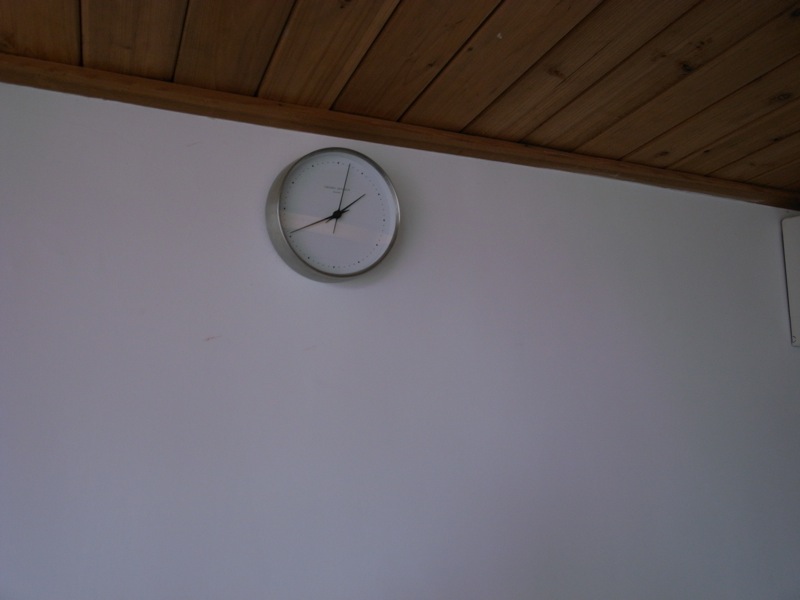The photograph captures a high-contrast interior scene featuring a round silver clock prominently mounted on a stark white wall. The clock's face is white with black hands, slightly off from 2:02, and is encircled by a brushed silver frame about three inches thick. The minimalist design includes black dots in place of numbers and faint, illegible lettering above the clock hands. Positioned unusually high on the wall, the clock almost touches a wooden border that transitions into a ceiling composed of vertically arranged wooden planks. This wooden ceiling introduces a warm, brown tone that contrasts with the crisp white wall, creating a balanced and visually appealing composition.